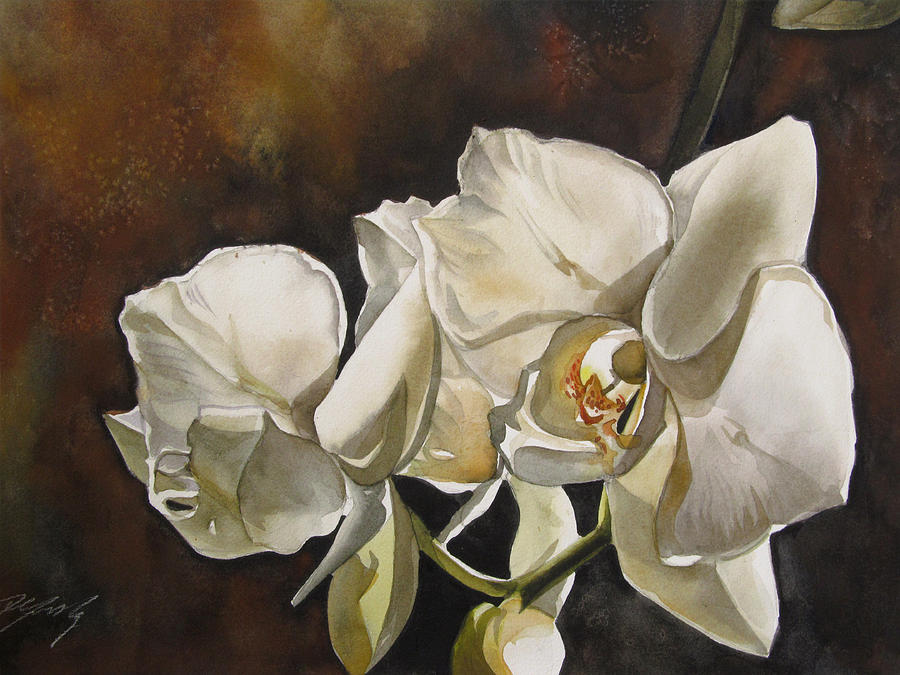The image showcases an abstract, artistic painting of two white flowers set against a variegated brown background. The painting employs a watercolor style, featuring subtle shading to indicate light and different shades of brown. The flowers themselves are predominantly white, with hints of cream, brown, and dark gray. The larger flower on the right is depicted face-on, revealing intricate details such as the orange pistil and a subtle hint of yellow, while the smaller flower on the left is shown in a side profile. Green veins branch from the bottom, leading into the blossoms, with at least one visible green leaf. A small, white cursive autograph is signed at the bottom left of the painting, adding a personal touch from the artist.